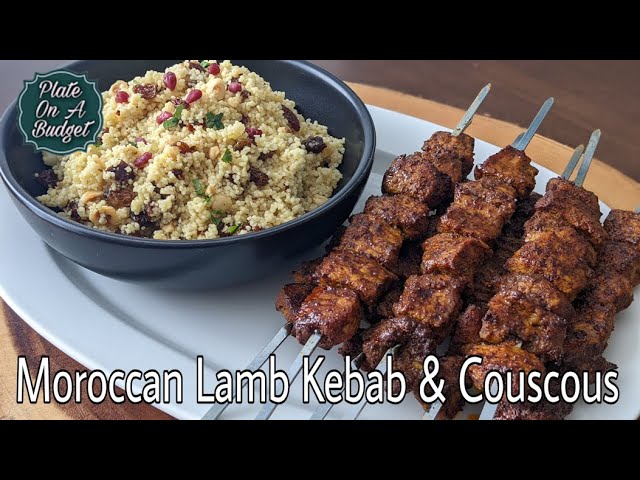The image showcases a vibrant and appetizing serving of Moroccan lamb kebab and couscous. At the bottom, the dish is labeled in bold, black-outlined and white-centered lettering. A logo in green and white, reading "Plate on a Budget" in tan color, is positioned in the top left corner. The culinary scene features a black bowl on the left filled with pale yellow couscous, adorned with colorful ingredients including red seeds, green herbs, and a hint of darker elements. To the right, juicy Moroccan lamb kebabs, arranged on silver skewers, display generous, succulent squares of meat, seemingly braised and grilled to perfection. These kebabs rest on a long, white serving plate, which is oriented at an angle, adding a dynamic visual element. The entire setting is brightly lit, capturing the detailed textures and rich colors with crystal clarity.